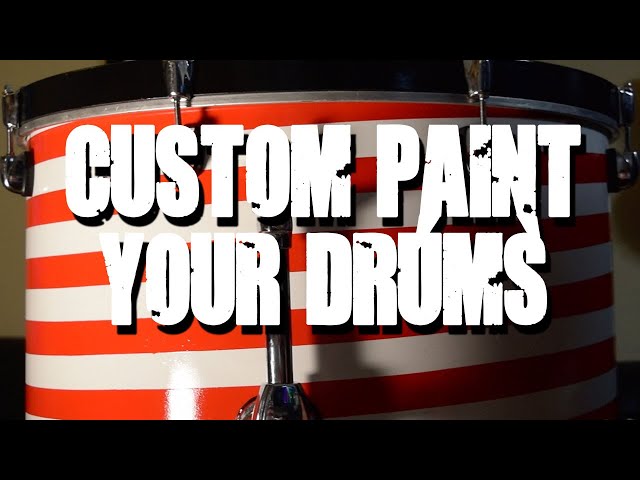In the center of this rectangular image, spanning about four to five inches wide and three to four inches high, there is a detailed view of a snare drum. The snare drum is primarily pale yellow in color and features horizontal red and white stripes on its exterior. It is framed at the top and bottom by black bars, each about half an inch in height, creating a moody and focused appearance.

At the very top edge of the drum, there is a black-painted rim. Surrounding the drum are various silver metallic components, including adjusters and bolts that secure the drum's structure. One notable feature is a metal bar running along the circumference of the drum's top.

The image is overlaid with bold white text that clearly states, "Custom Paint Your Drums," emphasizing the customization aspect visually promoted by the image's rich details and strong contrasts in colors and materials.